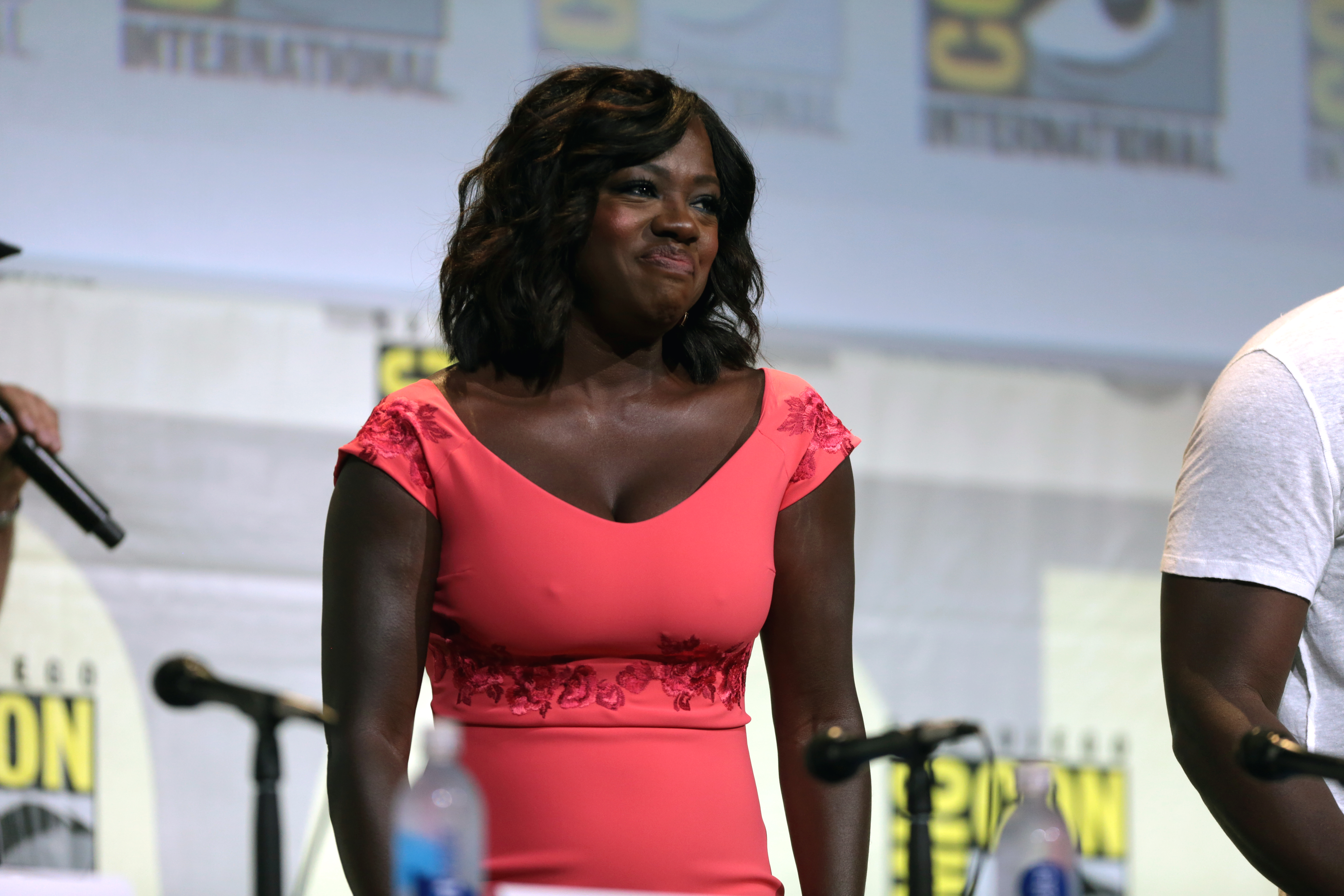In this photograph, a black woman with shoulder-length, wavy dark hair stands prominently. She is donning a coral-pink dress adorned with flower-like accents on the shoulders and around the waist. Her skin is a rich, dark brown, reminiscent of dark chocolate. The woman is positioned in front of a table set with microphones and a bottle of water, suggesting a press conference environment. To her left stands a black male in a white t-shirt. Behind the woman, a white wall decorated with Comic-Con posters can be seen.